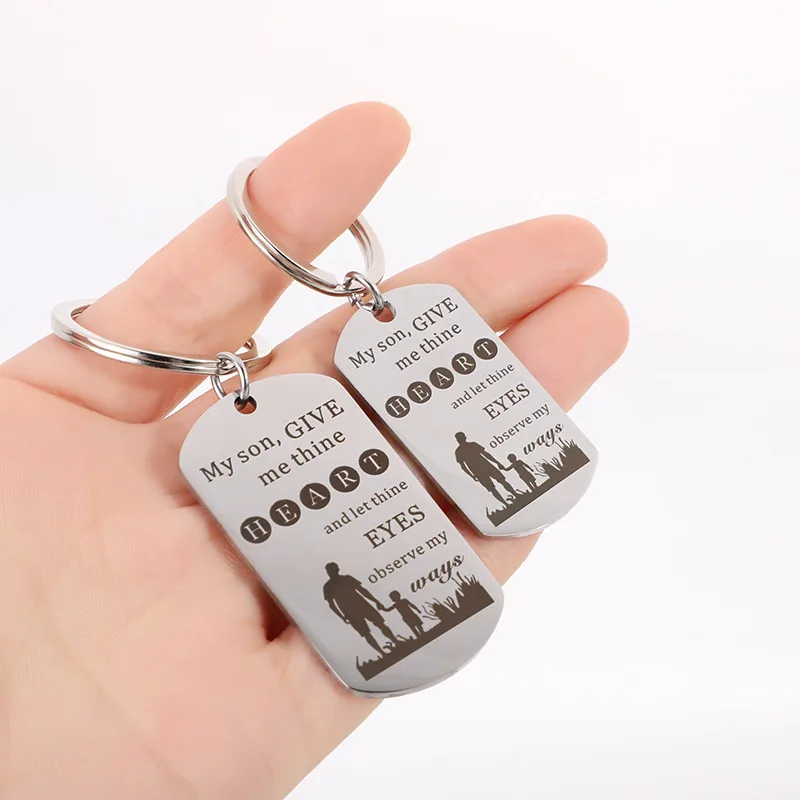In the photograph, a large, outstretched Caucasian right hand is shown palm-up, with only four fingers visible. The index finger prominently features two key rings, both silver and each holding a flat, dog tag-shaped plaque. These key chains are laid flat on the palm and angled slightly upwards. Each plaque has black engraving and displays the same text: "My son, give me thine heart and let thine eyes observe my ways." They also depict a silhouette of an adult man holding a little boy’s hand, walking through tall grass, with only the front view visible. The key rings are standard in thickness, unlike regular dog tags, and have rounded tops and bottoms with straight, angular edges. The plaques appear to be a heartfelt gift, possibly for Father's Day, symbolizing a father-son relationship.